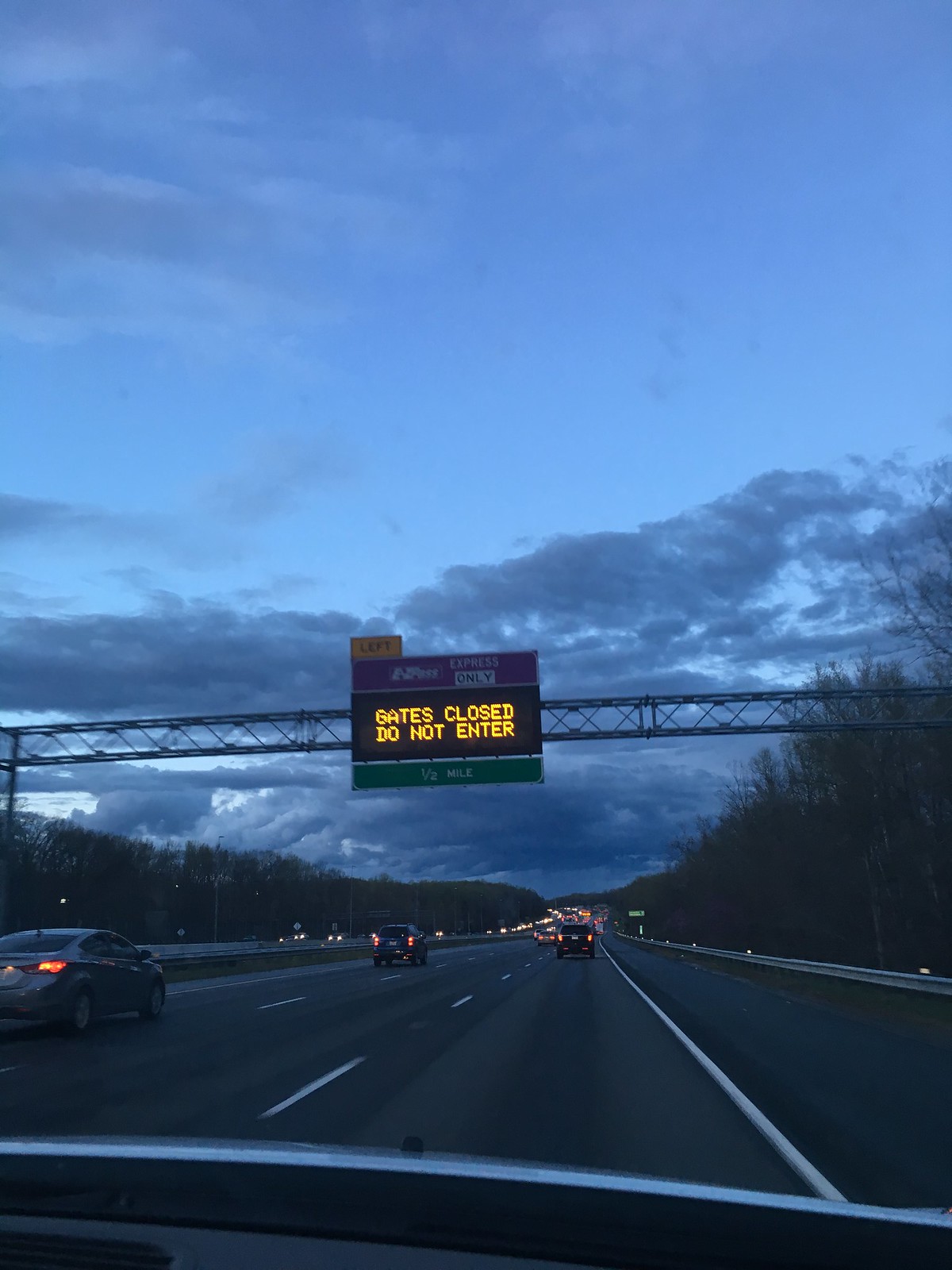A detailed photograph captures a highway scene taken from the front passenger seat of a moving car. The central focus is a prominent sign mounted on a horizontal metal structure above the freeway. This sign, comprised of a black display screen with bright yellow lettering, reads, "Gates Closed, Do Not Enter." Above this main message, in smaller text, the sign indicates directions with "Express" and notes a distance signifier of "Left, 1.5 Miles." The highway, extending straight from the bottom of the image up to about a third of its height, is flanked by dense trees on both sides. Several cars are visible on this side of the road, including two to the left of the photographer's vehicle and one directly ahead. The hood of the car the photo is taken from is slightly visible at the lower edge of the frame. To the left, the opposing lanes of traffic are congested with numerous vehicles. The image captures a sky that is light blue at the top and filled with gray clouds below, suggesting early morning or late evening lighting conditions.